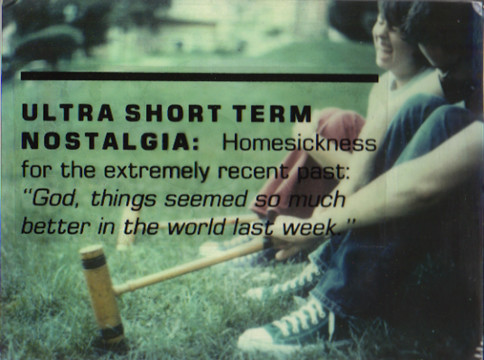This is a blurred and slightly out-of-focus photograph of two kids sitting beside each other on a green lawn, each holding croquet mallets. The girl on the left, dressed in red pants, is smiling with her eyes closed, seemingly laughing, while the boy on the right, also in Converse Chuck shoes, pulls his knees up with his arms wrapped around them, looking down. They both have blue Converse tennis shoes on. Overlaid on the photo in black lettering is an inspirational message that reads, "Ultra short-term nostalgia: homesickness for the extremely recent past. God, things seemed so much better in the world last week," capturing a sentiment of longing for better, simpler times.